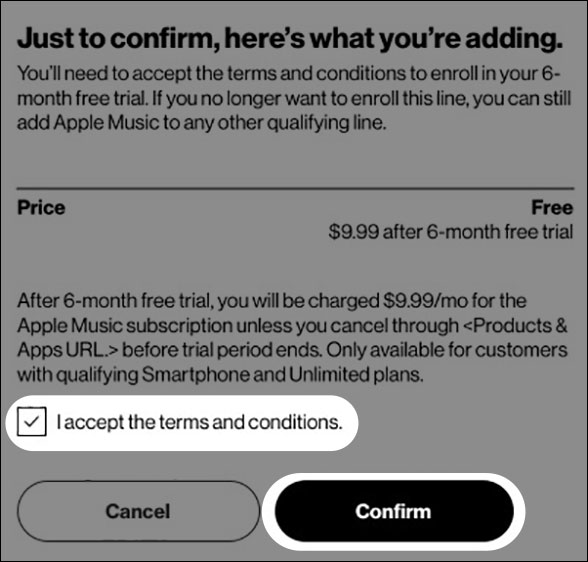The image depicts a subscription service agreement interface for Apple Music. At the top, there is a section with bold black text on a gray background that states, "Just to confirm, here's what you are adding." Users are prompted to accept the terms and conditions to enroll in a six-month free trial. It also mentions that if users decide not to proceed with this enrollment, they can still add Apple Music to any other qualifying line.

Below this text, a solid black line extends horizontally across the image. Further down, there is another section with the term "Price" in bold black text on the left and "Free" in bold black text on the far right. Underneath "Free," it states, "$9.99 after six-month free trial."

The subsequent text explains the subscription details: "After the six-month free trial, you will be charged $9.99 a month for the Apple Music subscription unless you cancel through the provided products and apps URL before the trial period ends. This offer is only available for customers with qualifying smartphones and unlimited plans."

At the bottom of the image, there is a white tab with a checkbox that reads, "I accept the terms and conditions." The checkbox is already ticked. Below this, there are two options: a "Cancel" tab and a "Confirm" tab. The "Confirm" tab is black with a white outline and has "Confirm" written in white text.